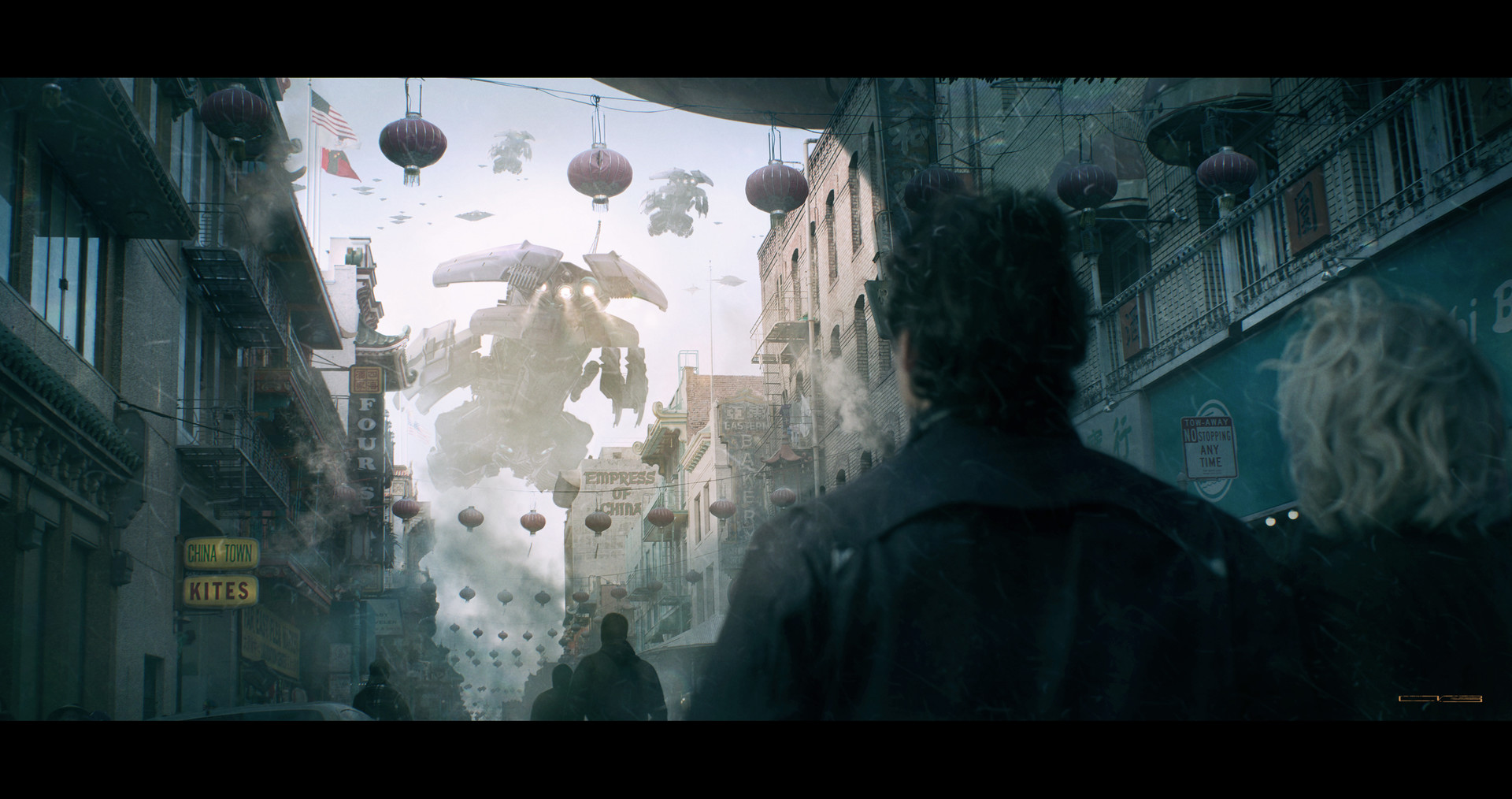The image appears to be a detailed still from a video game or sci-fi movie, displaying a scene filled with tension and curiosity. In the foreground, there are two figures—one a man with dark hair in a black jacket, and the other a woman with short blonde hair—both facing away from the viewer in the bottom right-hand corner. The setting is a bustling street in what seems to be a Chinatown, characterized by muted, grayish-blue tones and surrounded by three to four-story buildings. The building to the left features a yellow sign with the words "Chinatown" and "kites," and another sign mentioning "Empress of China."

Suspended between the buildings are large Asian lanterns, adding a traditional touch to the scene. Above them, the sky is filled with mechanical, bug-like flying machines emitting lights, resembling alien ships poised for an attack. These mechanical entities have arms and flood the sky with an eerie presence. In the background, the sky is tinged with sepia tones, further intensifying the sense of an ominous, sci-fi invasion. Smoke billows around the alien ships, suggesting chaos and destruction as they appear ready to assault the town, while the onlookers below gaze upward, seemingly unsure of what to make of the spectacle unfolding before them.